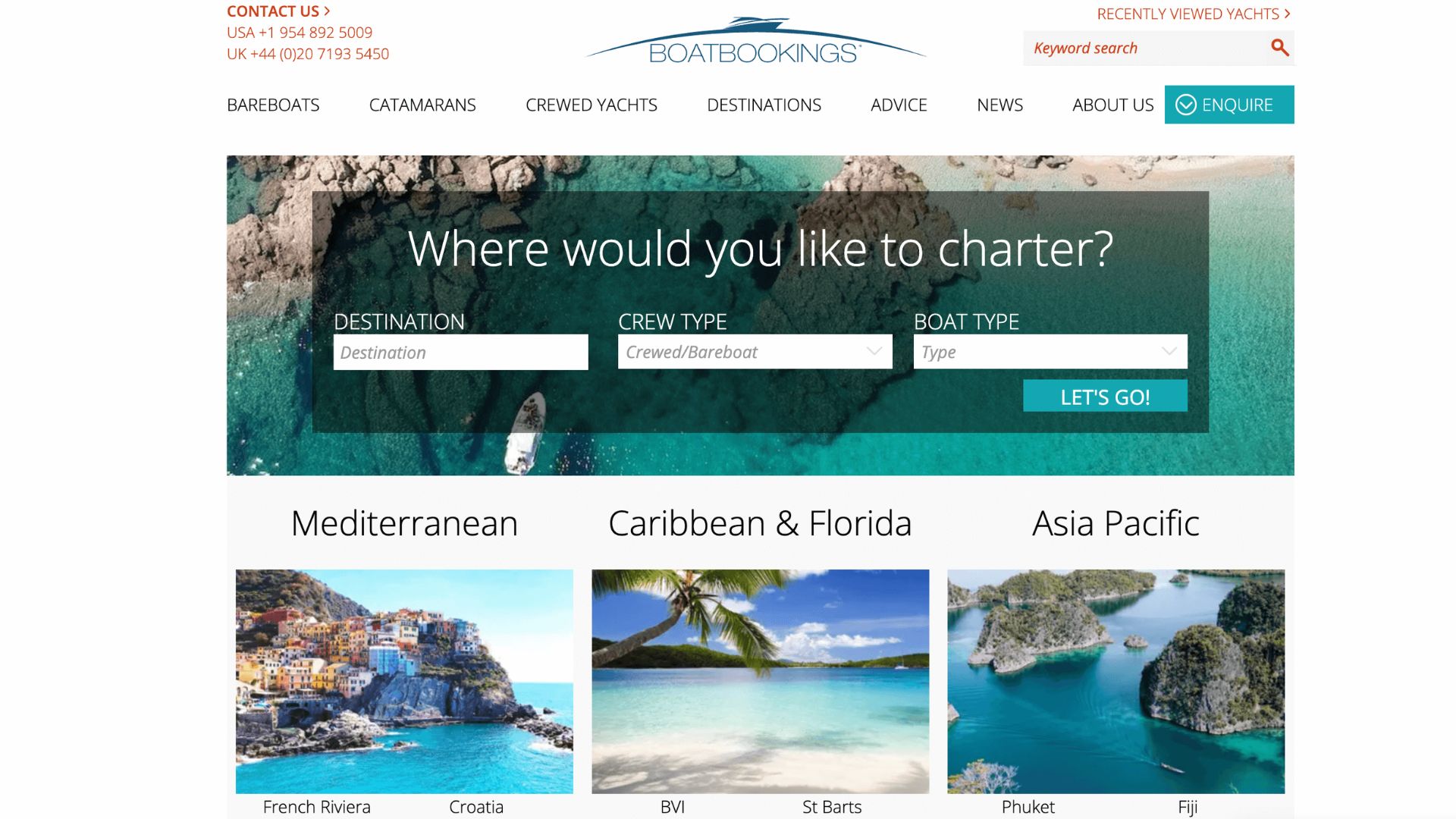This image is a detailed snapshot of a boat booking website. At the top left corner, contact information is provided: "Contact Us, USA: 1-954-892-5009, UK: +44 (0) 271935450". Centered, there is the website's title, "Boat Bookings," while on the right side, there is a section labeled "Recently Viewed Yachts." Beneath this title, users can type their queries into a "Keyword Search" field accompanied by a magnifying glass icon representing the search function. 

A navigation bar lies below, featuring links to various sections: "Bear Boats, Catamarans, Crewed Yachts, Destinations, Advice, News, About Us." To the far right of the navigation bar, there is a prominently displayed turquoise blue button labeled "Inquire" with white font.

The main image showcases an aerial view of a boat floating in crystal-clear, turquoise water, emulating a sense of tranquility and beauty. Overlaying this visually appealing scene is a semi-transparent gray rectangle containing a search form. This form prompts the user with the question, "Where Would You Like to Charter?" Below this prompt are three labeled fields: "Destination," "Crew Type / Boat Type," and "Boat Type." While the "Crew Type / Boat Type" and "Boat Type" fields feature drop-down menus, the "Destination" field is left as a text input. Finishing the form, a turquoise button labeled "Let's Go" encourages users to begin their search.